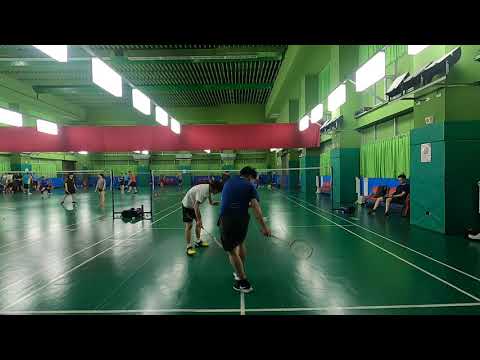The image depicts a large, bright indoor facility bustling with multiple teams engaged in what appears to be either badminton or tennis practice. The expansive space is predominantly green, with green ceilings, walls, and floors marked with white lines. Amidst the sea of green, a single red pipe runs through the scene. The central focus is on two individuals with dark hair; one is viewed from the back in a white t-shirt and black shorts, while the other, seen from the side, wears a blue t-shirt, black shorts, and black tennis shoes. Various groups are dispersed across the facility, each team on its own court, reinforcing the impression of a tournament or extensive practice session. An individual can be seen seated against the dark green wall to the right, adding to the sense of activity and preparation. The entire setting is well-lit by the bright interior lights, creating a vibrant and dynamic atmosphere.